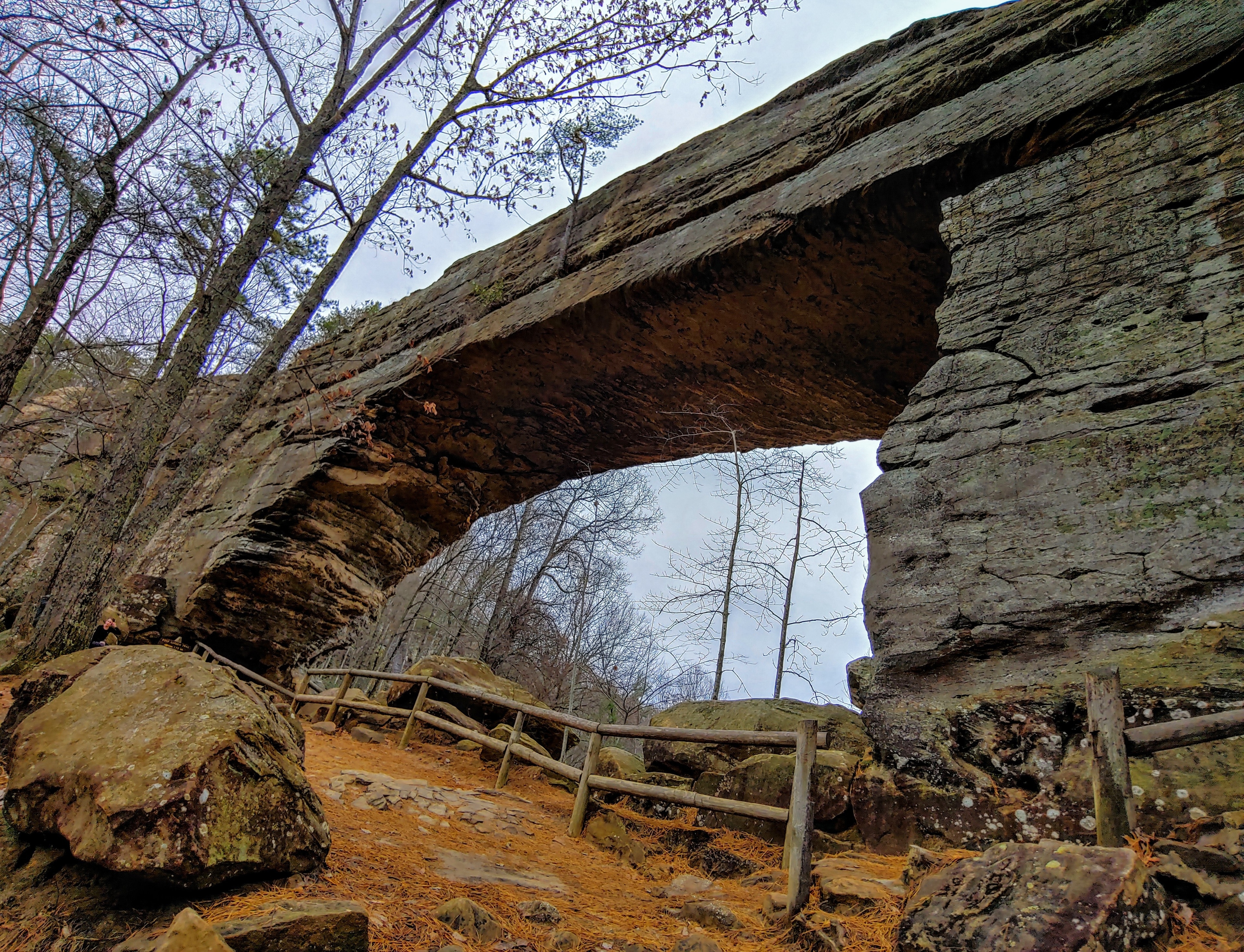A stunning natural stone bridge arches majestically across a wintery woodland scene, extending from the left to the right side of the image. This ancient formation, characterized by its layered, weathered appearance, hints at both natural erosion and the possibility of a previously complete rock wall now forming the bridge. The rugged bridge looks both sturdy and fragile, with cracks running through its surface and patches of green moss clinging to its crevices. Beneath the bridge, a rustic, broken-down wooden fence meanders through the landscape, seemingly guiding visitors along a path adorned with vivid orange moss and scattered stones.

Tall, leafless trees envelop the scene, their spindly branches reaching skyward against a backdrop of a partly cloudy blue sky. Some trees, tinged with remnants of autumn's red and brown hues, contrast with the brighter green foliage seen in the distance. A large brown rock anchors the bottom of the photo, adding to the composition's earthy tones of brown, gray, and black. The overall palette is rich with the colors of late autumn or early winter, painting a serene, slightly somber portrait of nature’s enduring beauty.